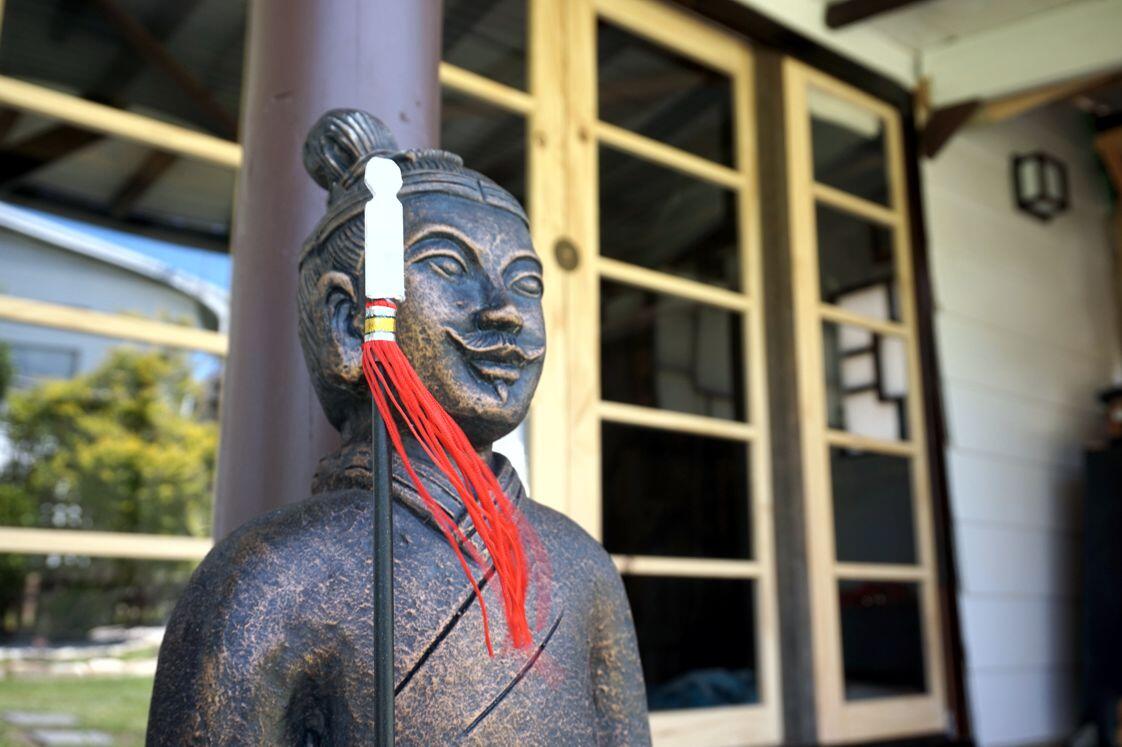This photograph captures a detailed image of a mini bronze or copper statue situated outside a building, positioned predominantly in the middle of the frame. The statue, displaying a dark brown to almost black hue with a subtle golden sheen, depicts a person with a pronounced facial structure, including full, slightly curled lips and prominent eyebrows. The figure sports a top-ponytail or a small circular bun on their head and appears to be a man, given the subtle mustache. The attire resembles a high-collared gi or a V-neck sweater, along with a sash detailed with lines down the front. The statue holds a black stick adorned with red tassels at one end and tipped with white at the other.

In the background, three light blonde wooden doors with tinted glass panes framed in five-square layouts are visible, reflecting a white house and trees to the left. A brownish-gray pole rises behind the statue, and a wall-mounted light fixture is discernible at the top right. This carefully composed scene blends the intricate details of the statue with the architectural elements of the building behind it.